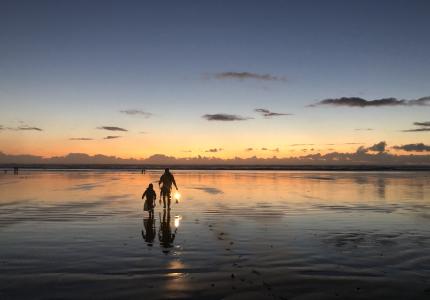The image showcases a serene beach scene at sunset, with the sky transitioning from deep orange and yellow near the horizon to darker shades of blue and gray above. In the center-left of the image are two silhouettes of people—a smaller child on the left and an adult to the right—walking along the damp, sandy shore where the receding tide has left behind smooth, wet sand marked with footprints. The adult holds a lit lantern in their right hand, casting a gentle glow around them. They appear to be carrying additional items, possibly for night crabbing or clamming, suggested by the buckets and wire mesh in their other hand. The distant horizon features a stretch of land beneath a line of clouds that stretches across the sky, with a faint afterglow of the set sun above the clouds. The peaceful scene is further enriched by subtle details like the wet sand reflecting the sunset hues, tiny ripples on the water, and some sparse beach vegetation. In the background, a few more people can be seen, indicating a shared activity, likely night fishing or clamming. The overall mood of the image is tranquil yet subtly dynamic, capturing the transition from day to night and the quiet activities of the beachgoers.